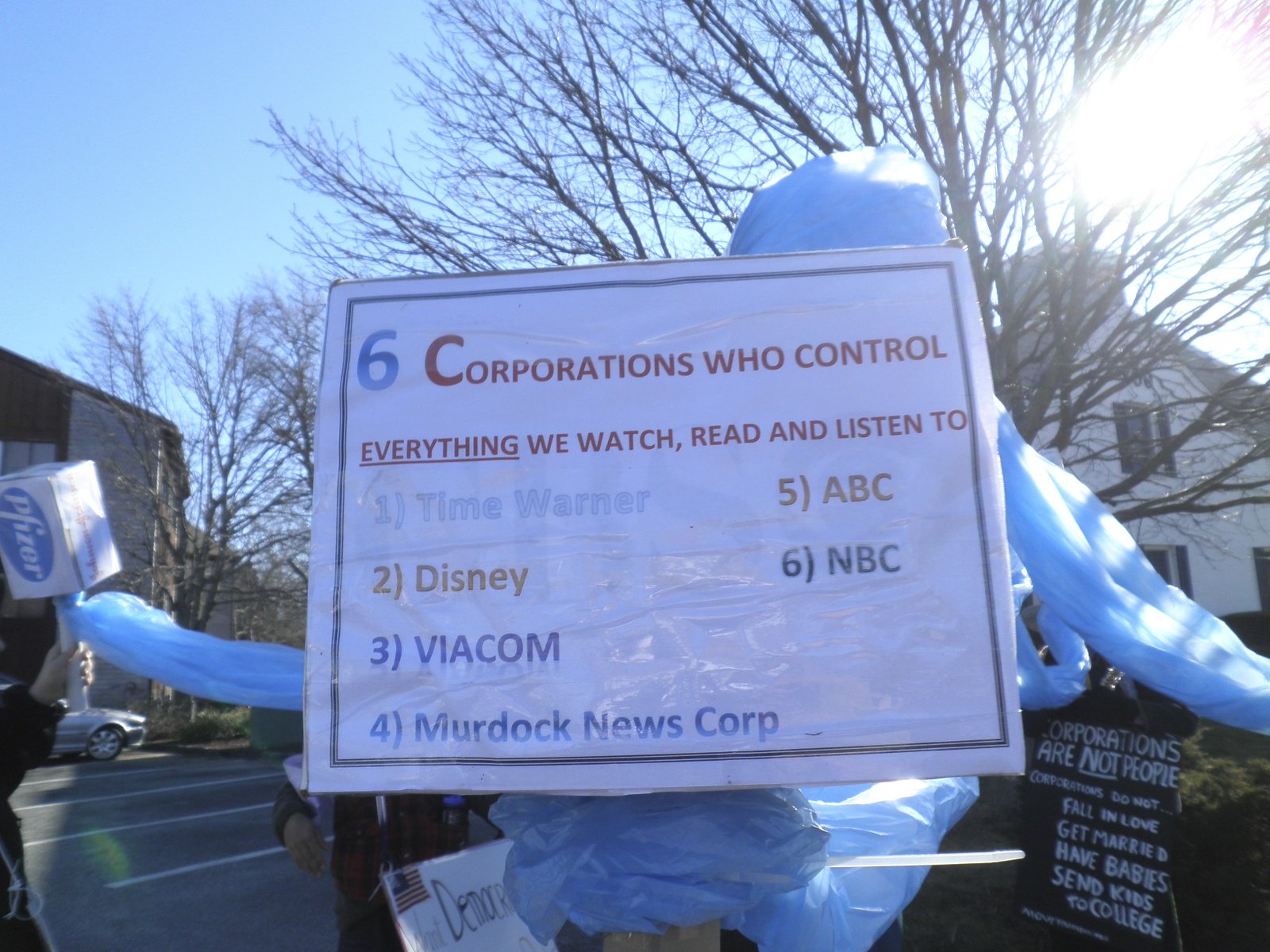The image depicts a protest scene set in a parking lot in front of a house. The area is strewn with trash and protest signs, prominently featuring messages against corporate influence. On the left side of the image, a hand holds up a box on a stick labeled "Pfizer." A laminated sign with a black border reads, "Six Corporations Who Control Everything We Watch, Read, and Listen To," listing Time Warner, Disney, Viacom, Murdoch News Corp, ABC, and NBC, with the text underlined in red. Another sign, handwritten, proclaims, "Corporations are not people. Corporations do not fall in love, get married, have babies, send kids to college." This sign is positioned at the bottom right, partially obscured by an American flag. A large, indistinct object looms in the background, and a leafless tree stands near a parked car, with sunlight visible behind the scene.